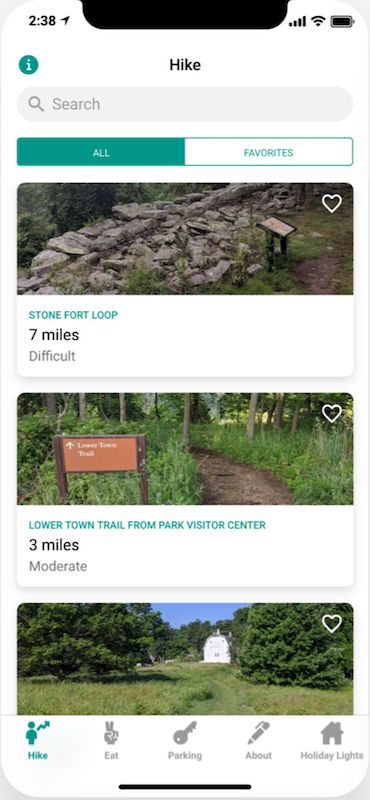This is a detailed screenshot from a mobile phone interface at 2:38, as shown in the top left corner. On the top right corner, cellular signal and a full battery icon are displayed. Centered along the top, the word "Hike" is written in black. Below the title is a rectangular search bar, and beneath that are two tabs. The first tab, labeled "All," features a green background, while the adjacent "Favorites" tab has a white background.

The main content of the screen includes three hikes, each depicted with an image and descriptive details. The first hike, titled "Stone Fort Loop," includes a photo of a stone structure and an adjacent directory. It is labeled as a difficult, seven-mile trail. The second hike, "Lower Town Trail from Park Visitor Center," is written in uppercase green letters and labeled as a moderate, three-mile trail. The image for this hike shows a dirt trail winding through a forest, and a sign in orange that reads "Lower Town Trail." The third image shows a barn amid abundant greenery, with trees and grasses surrounding it.

At the bottom of the screenshot, there are five icons representing different categories: hike, eat, parking, about, and holiday lights.